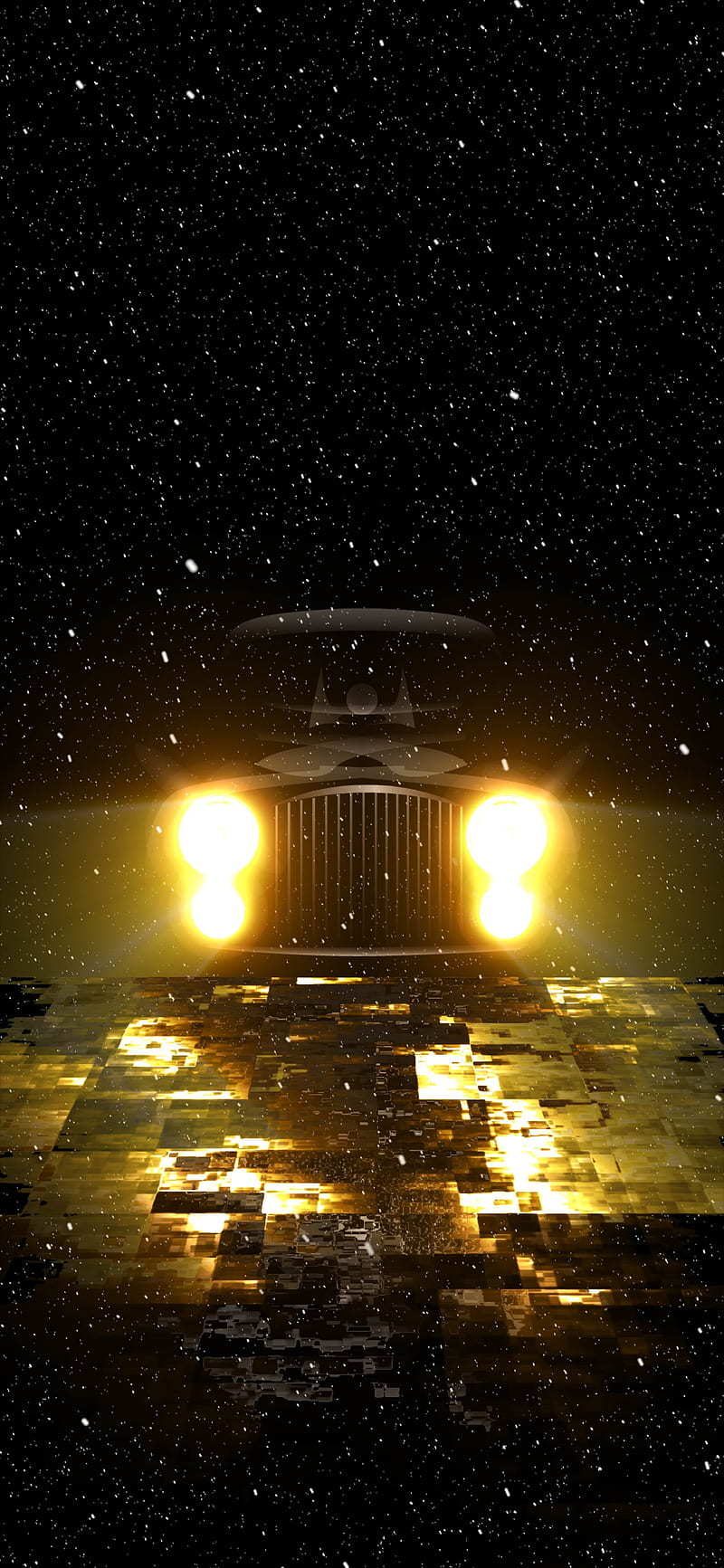In this striking nighttime photograph, a luxury vehicle, possibly a Rolls-Royce, faces the camera with its dual headlights illuminating the scene. The headlights, arranged with a larger light above a smaller one, create an intense glare, casting light onto the unusual, tile-like pavement below. The pavement is composed of interlocking tiles in various shapes and colors, primarily browns and creams, giving it a reflective, almost golden appearance. This tall, vertically-oriented image, much taller than it is wide, features a backdrop of an inky black sky filled with stars, giving the impression that the car is suspended in space. The car itself appears to be black, and its large, prominent grill stretches from the top of the hood down to nearly the pavement. The entire scene, devoid of any people or clear identifying marks on the car, is both ethereal and striking, with white flecks scattered throughout that resemble snowflakes, adding to the surreal and otherworldly atmosphere.